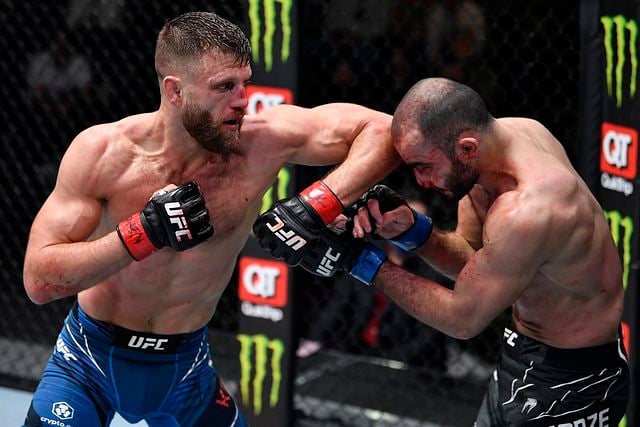A high-definition, horizontally-aligned rectangular photograph captures an intense UFC bout between two muscular, shirtless fighters inside a cage. The fighter on the left is mid-action, delivering a powerful elbow strike to the head of his opponent. He sports short brown hair, shaved sides, and a brown mustache and beard, showcasing his formidable build. He is adorned in blue shorts with "UFC" emblazoned on the waistband and "Crypto" visible on the side. His black gloves feature a white UFC logo, with distinctive red wrist cuffs. The fighter on the right, characterized by his partially bald head and short black hair on the sides, also has a black mustache and possibly a beard. He is defensively postured, head down and arms shielding his body, wearing predominantly black shorts with white UFC lettering. His gloves, similar to his opponent’s, bear the UFC logo but with blue wrist cuffs. The action takes place in a brightly lit arena with visible advertisements, including vertical neon Monster Energy banners and red squares with white "QT" for QuickTrip, adding to the dynamic atmosphere of the scene.